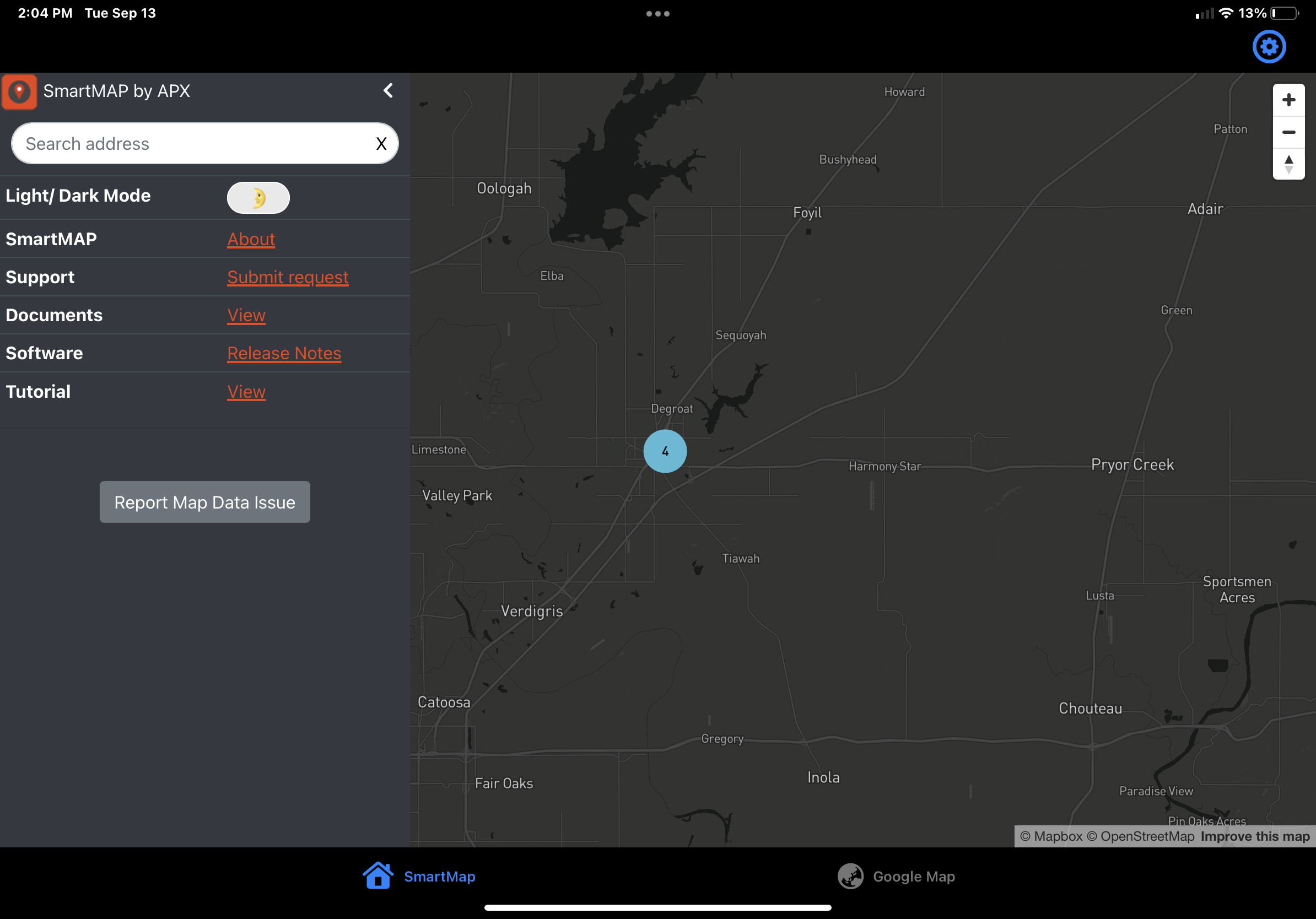In this detailed screenshot captured at 2:04 PM on Tuesday, September 13th, a variety of UI elements and map details are visible. At the top left, the timestamp is displayed in white text. The top right corner shows crucial status icons: an almost empty battery at 13%, a full WiFi signal, and a phone signal strength indicating only one bar.

The center of the image features a sophisticated map, possibly sourced from a website, presented in dark gray with black highlights. Prominent roads and locations are marked, with darker areas suggesting water bodies. One notable label, "Pyra Creek," appears on the far middle right of the map.

On the left side, a vertical rectangular box is present. At its top left, "SmartMap by APX" is prominently displayed in white text. Below this, an oval-shaped search bar invites users to "Search Address." Additionally, several features are listed: Light Mode, Dark Mode, SmartMap, Support, Documents, Software, and Tutorial, indicating a range of functionalities available for user interaction.